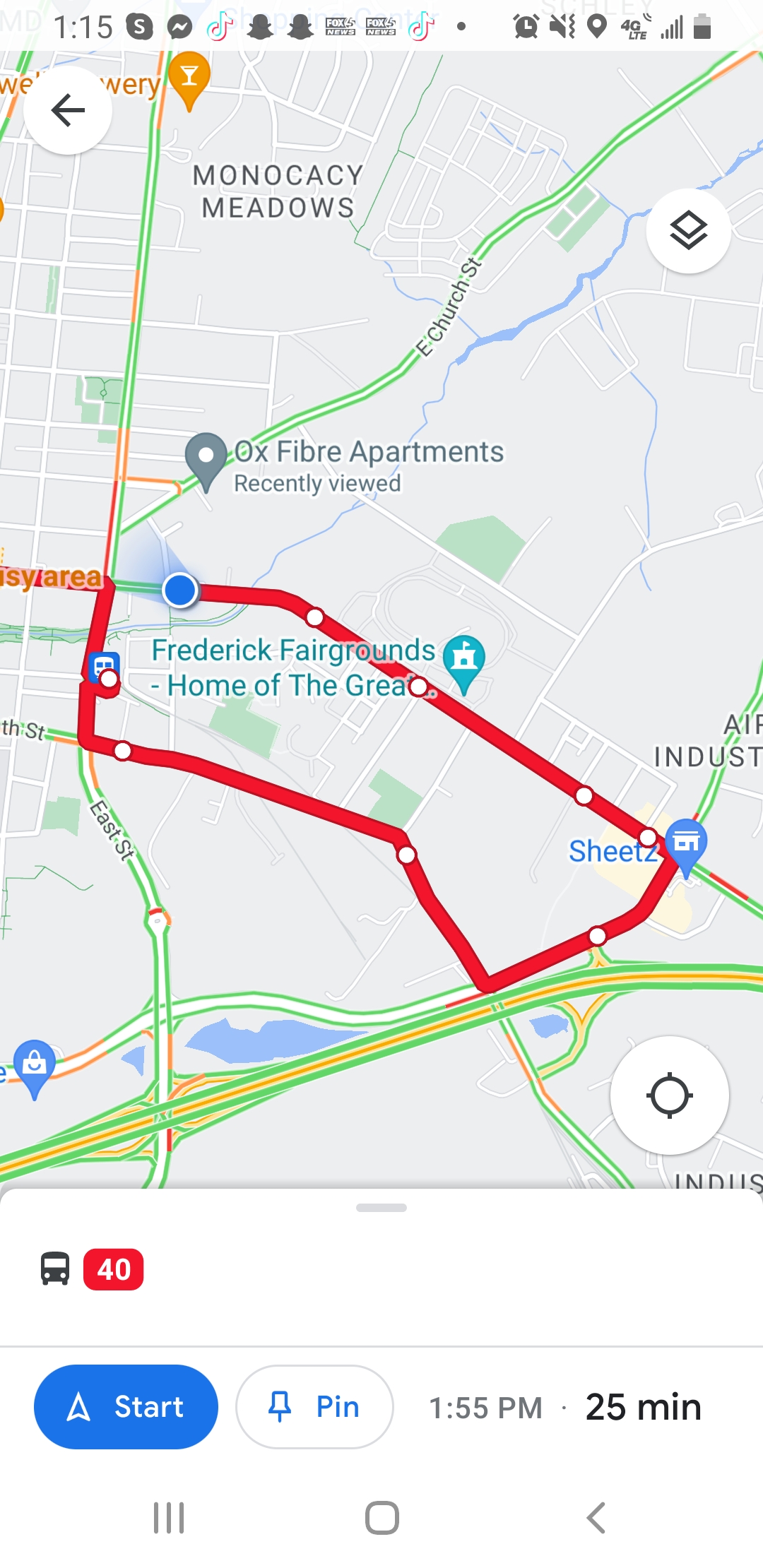This screenshot, taken on an Android device, displays a Google Maps screen with the interface showing various notifications at the top, including TikTok and Snapchat alerts, as well as indicators for muted volume, 4G connectivity, a half-dead battery, and the time, 1:15 PM. The main screen shows a set of directions highlighted in red—a common indicator for heavy traffic or delays—possibly due to an event at a venue called Frederick Fairgrounds, Home of the Great. The map pinpoints the current location with a blue dot and plots a red route winding past landmarks such as Monocracy Meadows, Oxfiber Apartments, Sheetz, and a bus stop, before continuing along a highway. The directions show options for travel: a 25-minute drive or a 40-minute bus ride, highlighted by a bus icon and a red lozenge displaying '40'. The interface includes a prominent blue 'Start' button for navigation, a pushpin icon labeled 'Pin', and indicates the time as 1:55 PM. The layout suggests that this route is situated in a suburban area just outside a city.